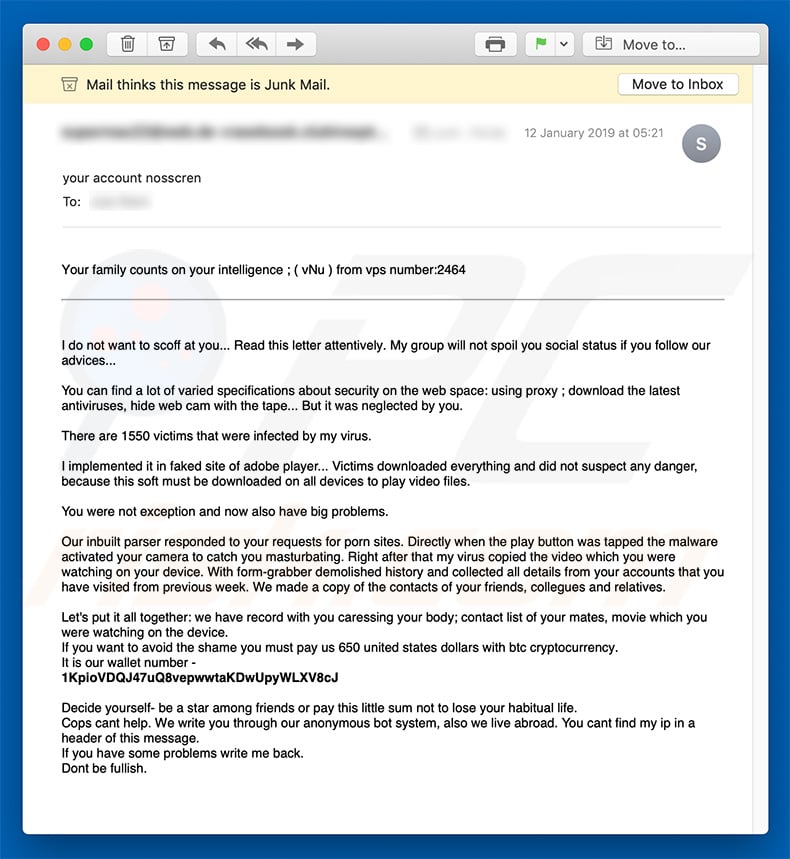The image is a vertical rectangle featuring a screenshot from an email program or app. The entire frame is bordered in blue. At the top of the image, there is a horizontal gray banner displaying several icons from left to right: a red dot, a yellow dot, a green dot, a trash can icon, an upload icon, a back arrow, a double back arrow, and a forward arrow. On the right side of this gray banner, there is a print icon, a flag icon, and a move to button.

Below this gray banner is a narrow horizontal strip in light yellow, indicating that "Mail thinks this message is junk mail," with a button on the right that says "Move to Inbox."

Further down, the email's date is shown as 12th of January 2019 at 5:21. The contents of the email appear to be suspicious, reinforcing its classification as junk mail. The email starts with "Your account, N-O-S-S-C-R-E-N, two," but this part is blurred out, likely for privacy. The message contains ominous and poorly written content, suggesting it is from a scam group. It reads: "Your family counts on your intelligence. I do not want to scoff at you. Read this letter attentively. My group will not spoil your social status if you follow our advices." The poor grammar and threatening tone further indicate the email's junk status.